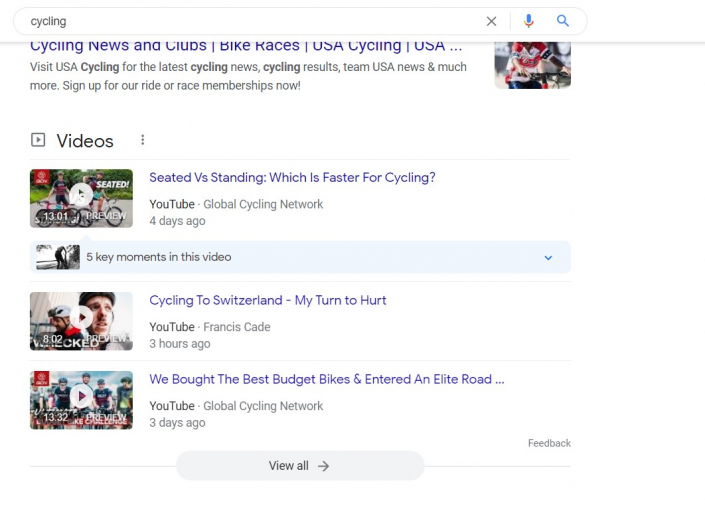A screenshot from a Google search for "cycling" captures multiple website and video hyperlinks. Most hyperlinks have titles in purple, indicating they have been previously visited by the user. The top result is for "Cycling News and Clubs," specifically focusing on bike races in the USA, accompanied by an image. Below this, there is a section titled "Videos," showcasing three YouTube videos. The first video, 13 minutes long, titled "Seated vs. Standing: Which is Faster for Cycling?" features an image of two cyclists riding side by side. The second video is titled "Cycling to Switzerland: My Turn to Hurt." The third video, recent content from the Global Cycling Network, is called "Rebought the Best Budget Bikes and Entered an Elite Road," uploaded three days ago. For comparison, the first video in this section was uploaded four days ago, while the second was uploaded just three hours prior to the screenshot being taken.